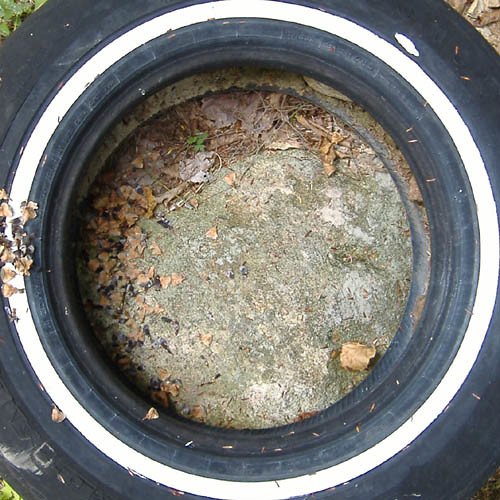The photograph captures an overhead view of an old, worn tire lying on a concrete floor scattered with brown and green leaves. The black tire features a singular white circular stripe at the top, framing a brown-toned surface within. The tactile details of the tire's wear and tear indicate that it may belong to a compact sedan rather than a larger vehicle. Surrounding the tire, brown leaves are prominently visible on the left side and in the corners of the image, adding to the scene's sense of neglect. The green leaves in the top left further contrast the decay, emphasizing the tire's age and disrepair.